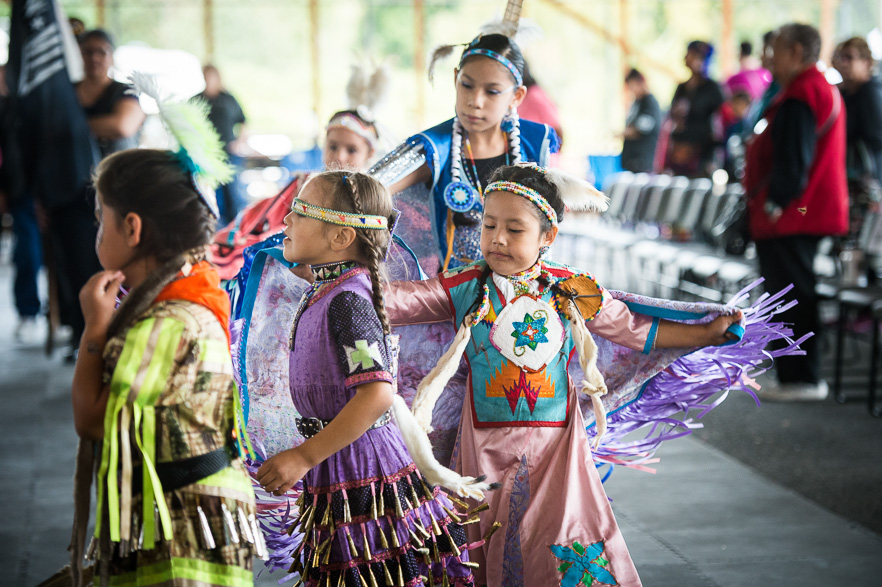The photograph captures a vibrant scene of young children, primarily girls, dressed in colorful, traditional attire that may be of Native American or Mexican origin. Their dresses are adorned with bright colors such as purples, pinks, and greens, featuring various intricate designs. The girls, likely participating in a dance performance, wear beaded headbands and ribbons in their braided hair, some ending in feathers. They are engaging in a dance, waving their dresses as they move in a circle, arms outstretched. 

In the foreground, three younger girls are aligned towards the left, with an older girl positioned behind them. The background reveals a group of adults standing around, observing the performance, as well as a row of chairs; the first row remains empty while subsequent rows are occupied. On the upper left side, a flag is partially visible. The environment suggests an open space with some structural elements, such as windows or exposed studs, and the flooring is a plain gray.